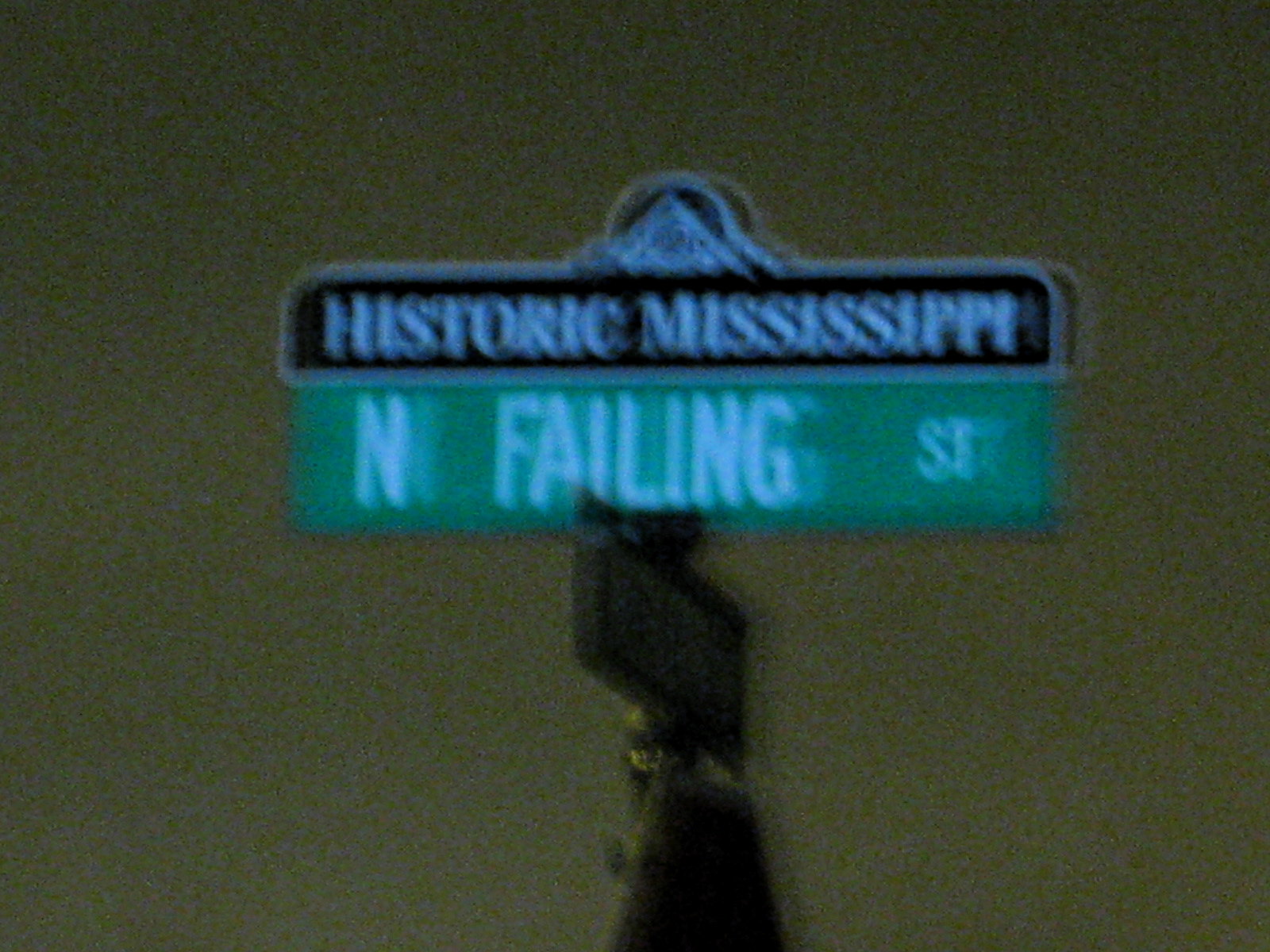The image depicts the top portion of a post situated on North Phelan Street, captured in an extraordinarily blurry photograph. The primary focus is on the North Phelan Street sign, which is a standard green road sign with "North Phelan" written prominently in white letters. The background is heavily blurred and predominantly olive green, rendering it unidentifiable. Above the North Phelan sign, another darkened, illegible sign marks a perpendicular road. Additionally, atop the post, there's a small, black plaque featuring white lettering and an illustration of a mountain, beneath which a slight bulge bears the inscription "Historic Mississippi," indicating the street's historical importance.